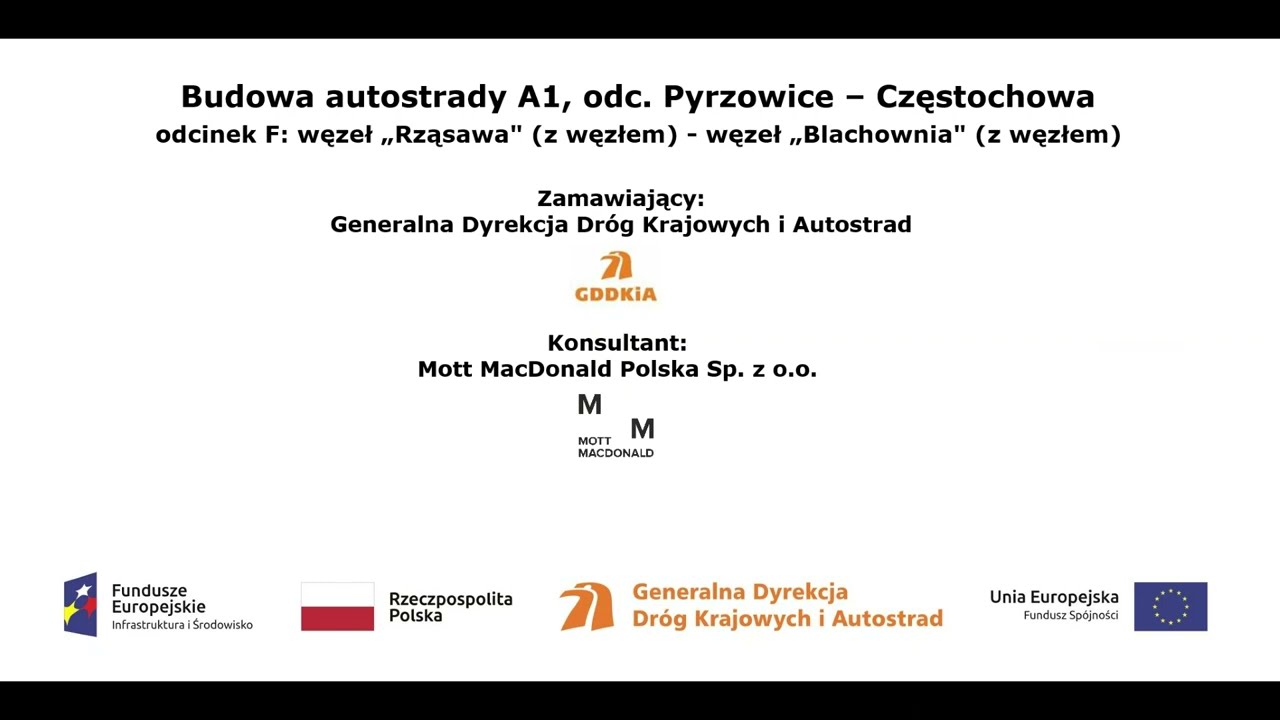The image features text predominantly in a non-English language, with key information presented against a white background. At the top, bold black text reads: "Budoa Autostradi A1,ODC period PYRZOWICE-CZESTOCHOWA." Beneath this heading, additional black text provides further details.

Centrally located in the image is more black text, written in another language. 

At the bottom of the image, a series of logos and flags are displayed from left to right. The first logo is a blue rectangle adorned with yellow, white, and red stars, accompanied by the text "FUNDUZE EUROPEJYSKI." Next to it is a flag consisting of two horizontal stripes, white on the top and red on the bottom. Following this is an orange logo that resembles a bird's head. Finally, the last emblem is a blue flag featuring a circle of stars.